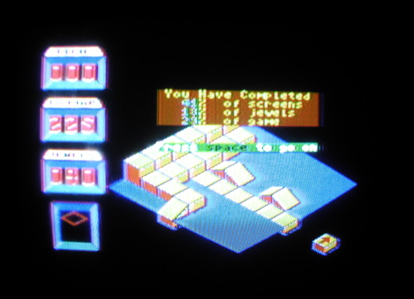This image appears to be a detailed screenshot from a retro video game. The background is black, and the central focus is a blue square, oriented like a diamond, filled with various white blocks. Some of these blocks have red, yellow, or orange sides, while others form triangular or stacked cube shapes. In the middle of the blue square are white shapes arranged in rows and columns, with one particular cube featuring an arrow. Overlapping this main diamond is a green stripe adorned with blue lettering and white symbols.

On the left side of the screen, there are four vertical blue rectangles that extend into the background. Each of these rectangles contains three red shapes, varying slightly in design, and the bottom rectangle uniquely features a red diamond. Above the blue square is a brown rectangular box with yellow text that reads, "You have completed this many screens, this many jewels," followed by another term left ambiguous. Blue numbers intermingle with the gold text, providing specific counts or percentages. The entire composition suggests the player’s progress or achievements within the game.